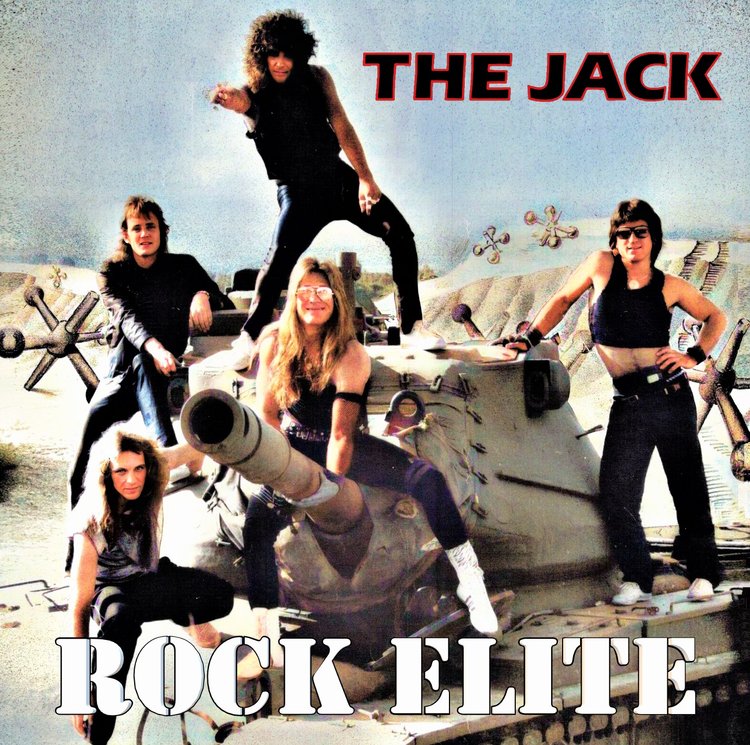The album cover for "The Jack" by Rock Elite features a striking World War II-themed photo with a khaki military tank as the focal point. Five band members, embodying the classic 1980s big hair rock style, are positioned around the tank. One member with long black hair, dressed in all black, stands on top of the tank pointing towards the camera. Another, also with long black hair and dressed in black, leans against the side of the tank. Kneeling nearby is a third member wearing a gray shirt and black pants. A fourth band member straddles the tank's cannon, donning sunglasses, blue jeans, and white tennis shoes. The fifth member, with long black hair and in dark clothing, stands near the cockpit area. Scattered throughout the scene are old metal jacks, adding a whimsical touch. The album title "The Jack" appears in the top left in bold black letters outlined in red, while the band name "Rock Elite" is displayed across the bottom of the tank in white text with a black outline.